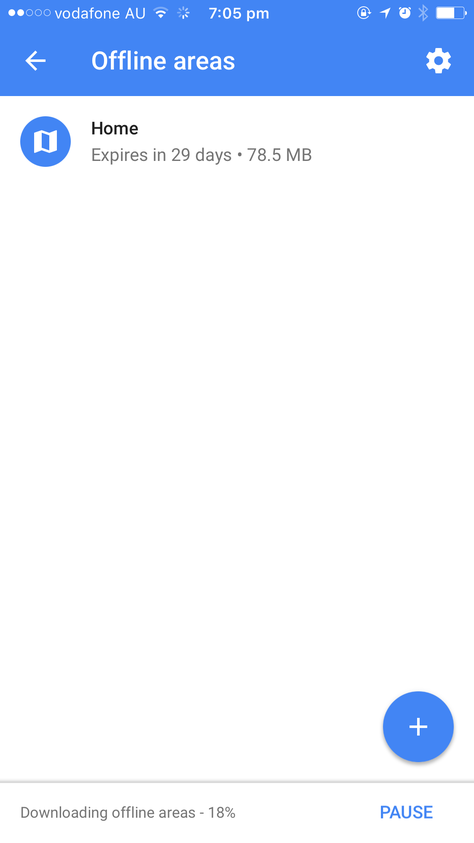The image appears to be a screenshot from a smartphone. At the very top, there is a rectangular blue box showing two white dots followed by three circles. The text "Vodafone AU" is displayed, indicating the mobile network provider. Next to it are icons showing signal strength, operational status, the time "7:05", and the battery life on the left side. Also on the left is another signal strength indicator. 

Beneath this blue box, there is a left-pointing arrow labeled "Offline areas". On the extreme right of the blue box, there is a settings icon. 

Below this section, there's a blue circle containing an open box icon with the text "Home" written in black letters. The next line reads "Expires in 29 days" and shows "78.5 MB". 

Towards the bottom of the image, there is a blue circle with a plus sign, followed by a gray progress bar indicating that "Offline areas" are being downloaded at 18%. Beside the progress bar, there is a blue pause button.